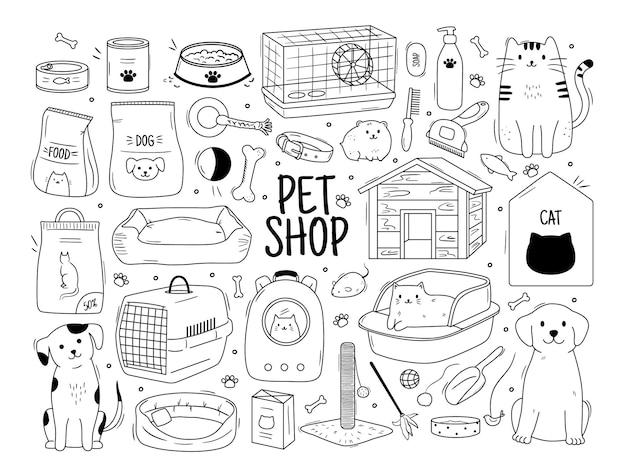This detailed black and white illustration depicts a lively and bustling pet shop scene. At the center, bold black letters spell out "pet shop," surrounded by a vast array of pet-related items. The lower left and lower right corners feature stylized, happy-looking dogs with joyful expressions, while the upper right corner showcases an equally content cat. The entire illustration is filled with intricate drawings of pet supplies, including various food bowls, pet toys, a hamster cage with a wheel, a cat carrier, a dog house, and a variety of grooming tools such as brushes and soaps. There's a distinctive backpack with a plastic window, designed for pets to look out, and an assortment of other items like toy fish, collars, and beds for both cats and dogs. Additionally, the top left corner highlights a can of tuna and a dog bone, with a can of dog food and more pet supplies scattered throughout. This image, likely computer-created, features each item meticulously outlined in black against a white background, resulting in a vibrant and detailed portrayal of a well-stocked pet shop, appealing particularly to children.